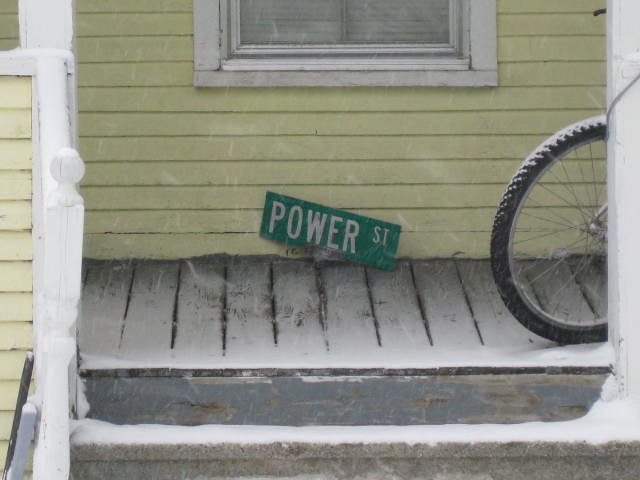The photograph captures a worn wooden front porch of a pastel yellow clapboard house on a low-light day. The steps leading up to the porch, partially dusted with snow, are bordered by a white railing and a white post. The paint on the steps, once a dark grey or bluish-grey, is chipped and faded. The bottom edge of a window, trimmed in white, is visible, adding contrast to the yellow exterior of the house. On the porch, a green street sign with white lettering reads "Power Street," lying in the center. To the right, there is a partial view of the back tire of a bicycle, also dusted with snow. The photograph presents a scene devoid of people, animals, and vegetation, emphasizing the aged and weathered elements of the house.